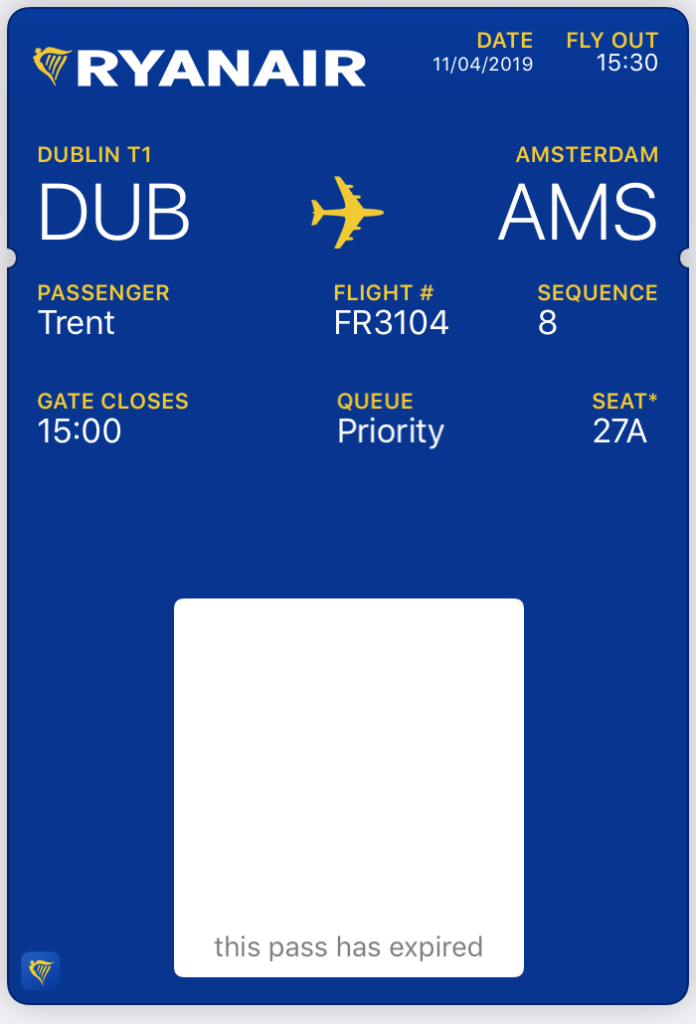A detailed visual representation of a Ryanair boarding pass is displayed on a blue background via the Ryanair app. The top left corner features "Ryanair" in bold white text beside the airline’s signature yellow logo. In the top right corner, the date "11-04-2019" is displayed, along with the departure time "15:30." Below these details, the flight information indicates departure from "Dublin T1 (DUB)" to "Amsterdam (AMS)" with a small plane icon signifying the route. Further down, the passenger’s name, "Trent," alongside pertinent details, such as "Flight Number: FR3104," "Sequence: 8," "Gate Closes: 15:00," "Priority: Q," and "Seat: 27A" are clearly listed. At the bottom, an important note reads, "This pass has expired," indicating that the boarding pass is being viewed post-flight. Overall, the image provides comprehensive details of Trent’s travel logistics for his flight from Dublin to Amsterdam, highlighting specific elements such as the sequence number and seating arrangement.